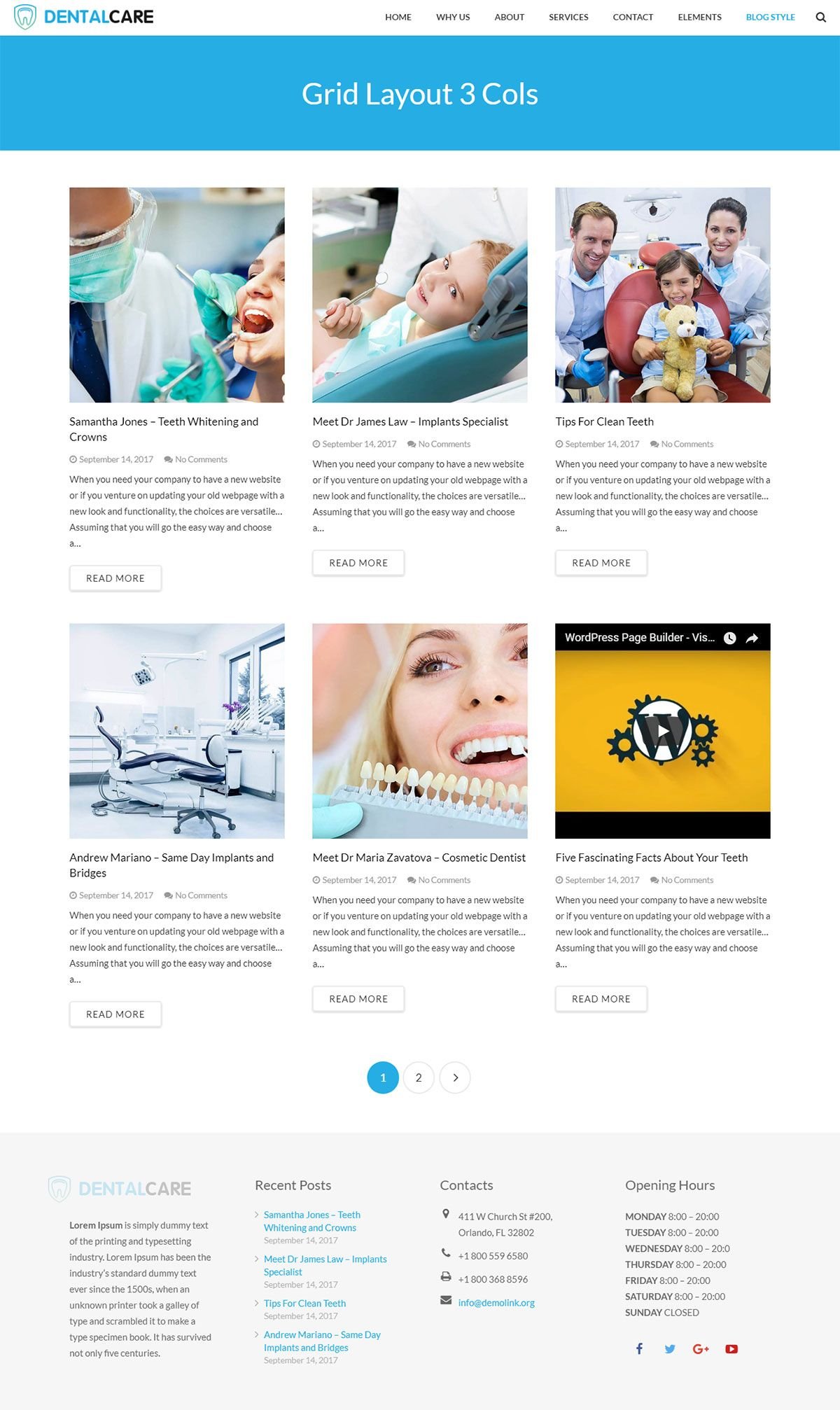The screenshot resembles a typical layout from a dental care website. At the top, there is a white header featuring the "Dental Care" logo — with 'Dental' in blue and 'Care' in black, accompanied by a tooth icon to the left of the text. To the right, in slightly smaller font, are navigation tabs labeled Home, YS, About, Services, Contact, Elements, and Blog Style, with 'Blog Style' highlighted in blue, indicating it is the current selection. A magnifying glass icon representing the search function is also visible.

Beneath this header, a solid blue banner appears with centered white text that reads "Grid Layout 3COLS." The main content section below the banner is organized into two rows, each with three images depicting various dental office activities. Each image has a brief descriptive text underneath, followed by the date and a comment section to the right. Below each description is the beginning of an article with a "Read More" button on the bottom left to access further information.

At the bottom of this section, there are navigation buttons for pagination — a '1' highlighted in blue, a '2', and a 'greater than' symbol encased in white circular icons, indicating multiple pages.

The footer of the website is presented in a gray rectangular format. It starts with the "Dental Care" logo again and some placeholder text. There are three distinct columns underneath: the first features recent posts with clickable links, the second provides contact information such as address, phone numbers, and an email address, and the third outlines the operating hours, detailing the daily schedule. At the lower right of the footer, social media icons for Facebook, Twitter, and Google+ are present, suggesting options for sharing or following the dental care website on these platforms.